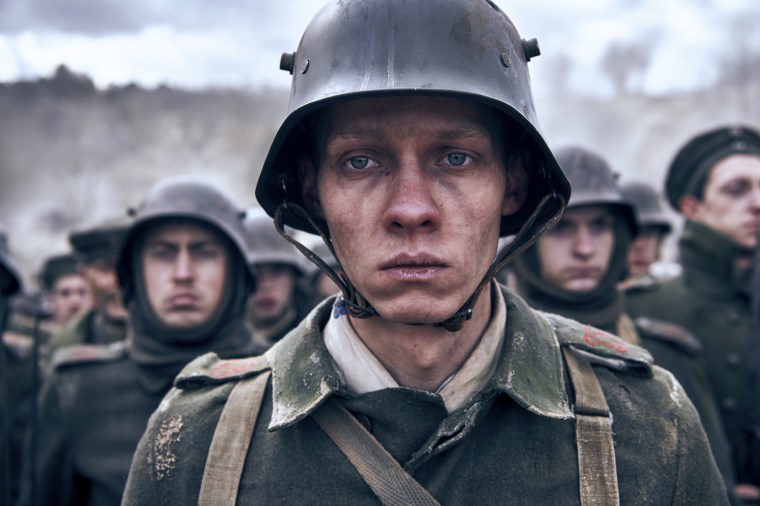The image appears to be a still from a World War II movie, capturing an emotionally charged moment. Front and center is a soldier wearing a distinctive, dark green German-style helmet, which may also resemble Soviet designs, adding ambiguity to his allegiance. His expression is one of utter defeat, sadness, and exhaustion, with dark lines under his eyes emphasizing his weariness. He stands directly facing the camera, almost soulless, with a heavy dark green coat and the straps of a backpack visible. Behind him, other soldiers line up, all dressed in similar uniforms, some with helmets and one notably with a hat. The background is greyed out and fuzzy, featuring indistinct trees and grass, contributing to the barren, lifeless feel of the scene. The overall mood is one of desolation and hopelessness, effectively conveying the hard realities of war.